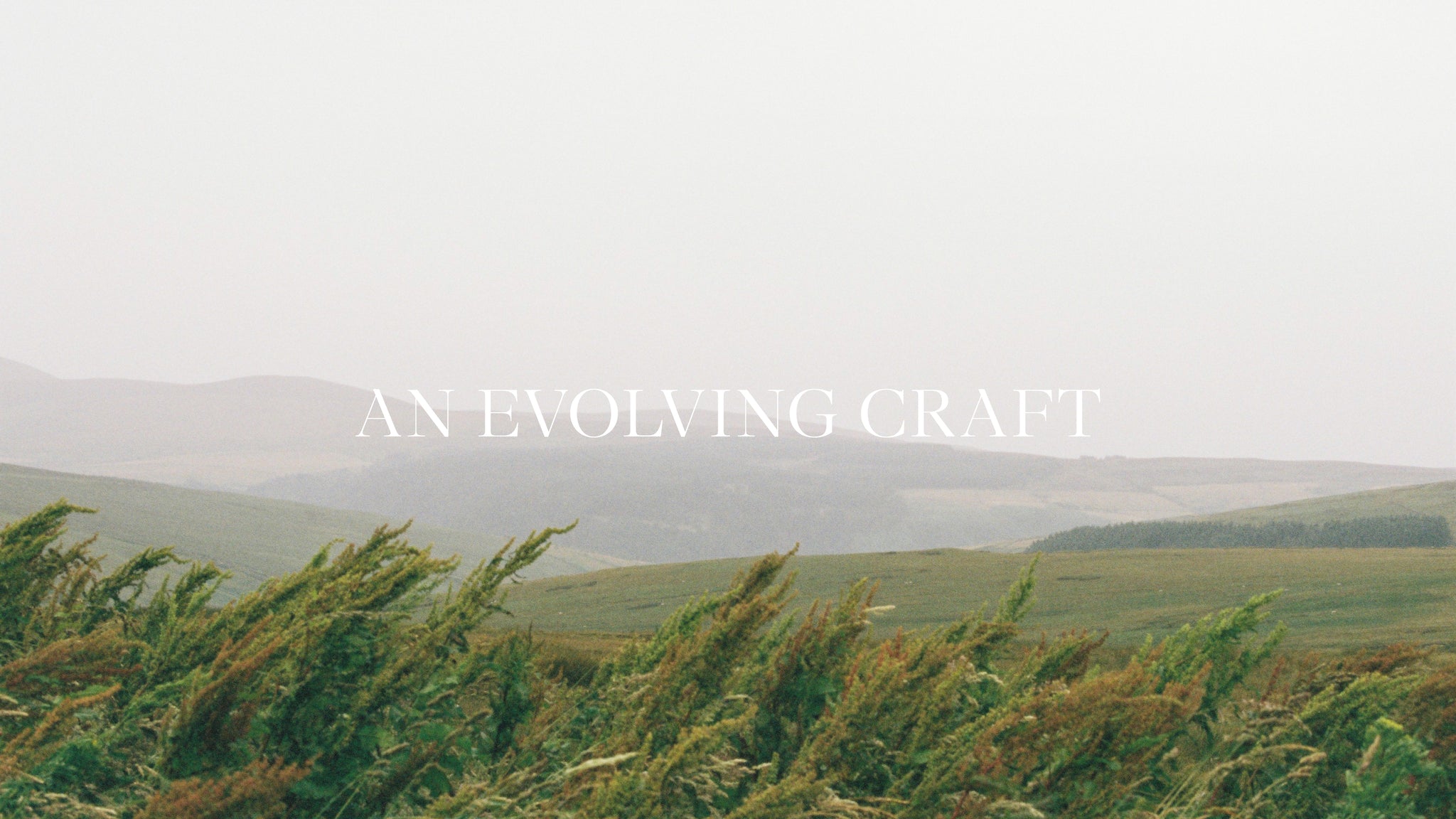The image, possibly a CGI or drawing, depicts a serene outdoor landscape with a cold vibe, reminiscent of the rolling green hills of Ireland. In the foreground, vivid green and brown grass and weeds, swaying as if blown by wind, lean from left to right. This leads to a flat brown patch of land, followed by a larger grassy area on the right. As the scene recedes, a small hillside rises on the left, while flatter grassy terrain and sporadic trees appear to the right. The middle distance reveals a valley-like area shrouded in fog, with shorter and taller hills scattered throughout, culminating in hills on the left and flatter land on the right. The entire scene is enveloped in a light gray sky, under which white uppercase text reads "AN EVOLVING CRAFT" across the middle of the image, positioned at the horizon of the farthest hillsides.